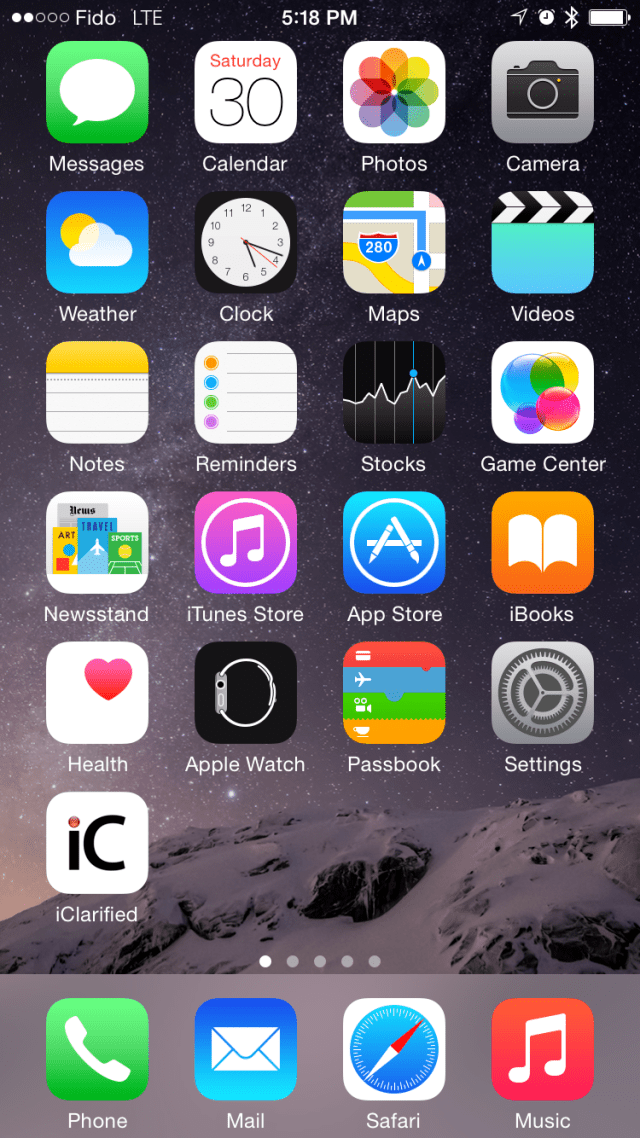This is a detailed screenshot of a smartphone home screen. The background image features a breathtaking view of snow-covered mountains under a starry sky. The screen displays several app icons:

1. **Messages** - A green tile with a white speech bubble icon.
2. **Calendar** - A white square displaying a red "Saturday" and "3-0" below it.
3. **Photos** - A white rectangle featuring the Photos app logo.
4. **Camera** - An icon of a camera.
5. **Weather** - A blue icon with a sun and cloud illustration, labeled "Weather" underneath.
6. **Health** - A white icon with a red heart, labeled "Health" in white text.
7. **Phone** - A green square with a white telephone icon, labeled "Phone" below.
8. **Mail** - A blue square with a white envelope icon, labeled "Mail" in white text.
9. **Music** - A red square with a white music note icon, labeled "Music" underneath.
10. **iBooks** - An orange square with the outline of an open white book, labeled as "iBooks."
11. **Apple Watch** - A black square with a watch icon, labeled "Apple Watch."

The arrangement and variety of the icons provide a glimpse into the user's frequently accessed applications against the serene and majestic mountain backdrop.